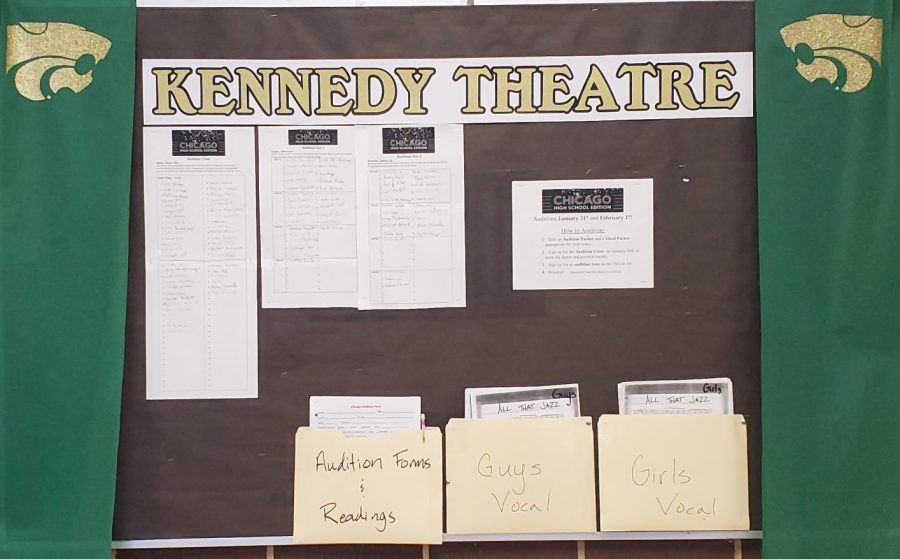The photograph, taken indoors using artificial light, showcases a horizontally rectangular bulletin board typical of a high school setting. The board's edges are adorned with green banners, each featuring a gold emblem of wildcats with their mouths open, facing each other. Dominating the center of the board is a brown-maroon section with a white, rectangular banner displaying the text "Kennedy Theater" in gold lettering. Below this banner, several white sheets of paper with the Chicago play logo, featuring black text and triangles, are pinned to the board. At the bottom, three bone-colored manila envelopes are affixed, labeled respectively as "Audition Forms and Readings," "Guys Vocal," and "Girls Vocal." Each envelope seems to be stuffed with papers. The overall color scheme is neutral, with accents of gold, maroon, brown, and green. Additional text on the papers is too small to read clearly.